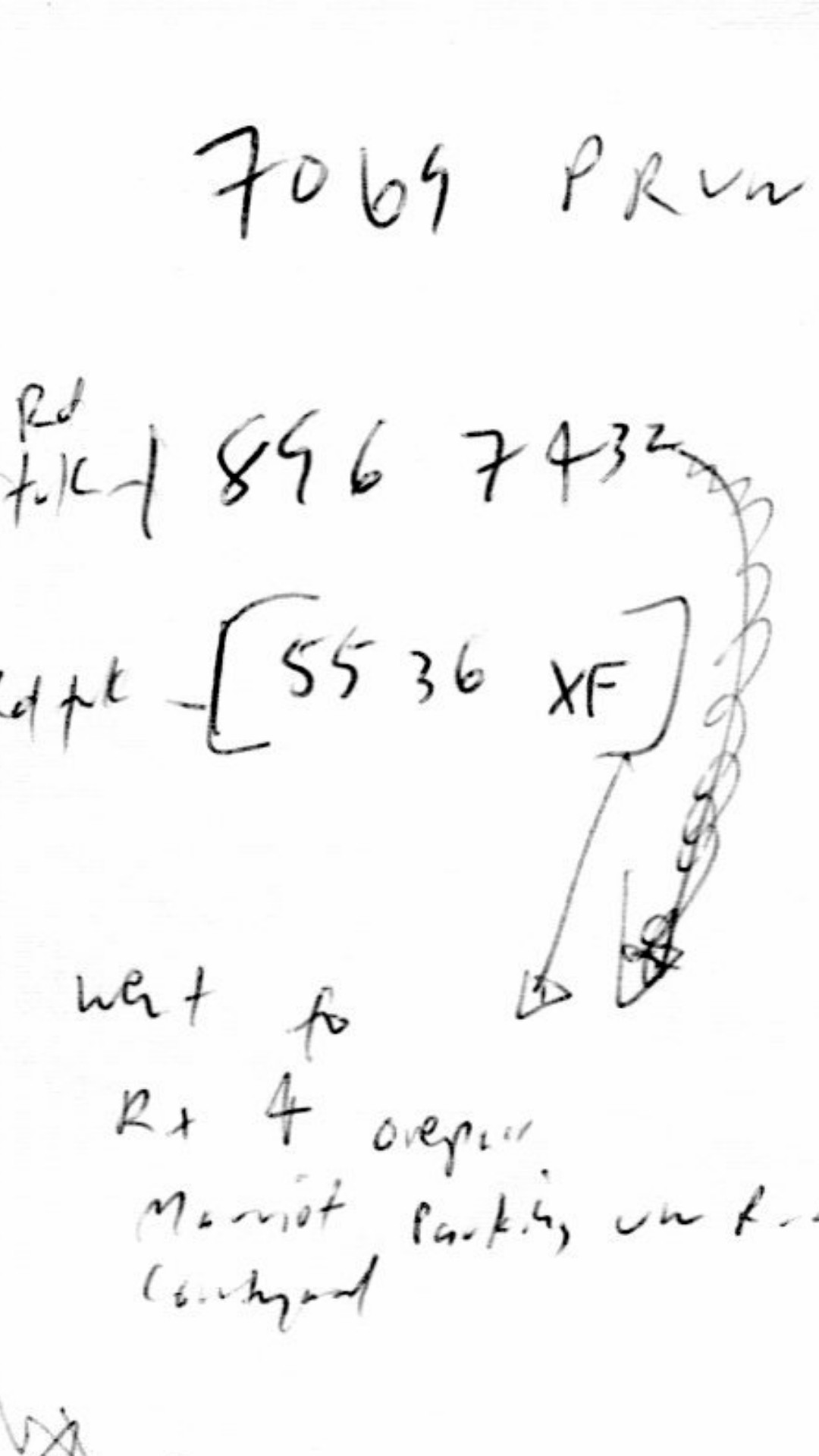The image showcases handwritten text on a white background, all penned in black ink. The first line starts with the number 765; however, the last digit is ambiguous and could be interpreted as an incomplete 9 or an S, rather than a 5. Following a space, there are the letters "PR" and then either a "U" or a "V", and a somewhat blurred "N" or "W", with the latter being more likely despite the faint left side.

Further down, towards the center, appear the letters "R" and "D" followed by "T", "U", "L", and a character resembling a "C" connected to a prominent vertical line. Below this are the numbers "896" and "743". Directly underneath these numbers lies "5536XF" enclosed in rectangular brackets. Some unintelligible text occupies the left side of the image.

To the right of the centrally placed numbers, there are arrows pointing downwards. The arrow extending from the right bracket of "XF" is straight and diagonally directed slightly leftward. Contrarily, the arrow stemming from "743" curves slightly and includes a squiggly line, indicating an attempt to scribble something off. Both arrows converge towards more indistinct text, where the first word might be "went", followed by "to", with the remaining words being unreadable.

Additionally, a faint symbol or possibly more text appears in the bottom left corner of the image, contributing to the overall enigmatic presentation of the handwriting.